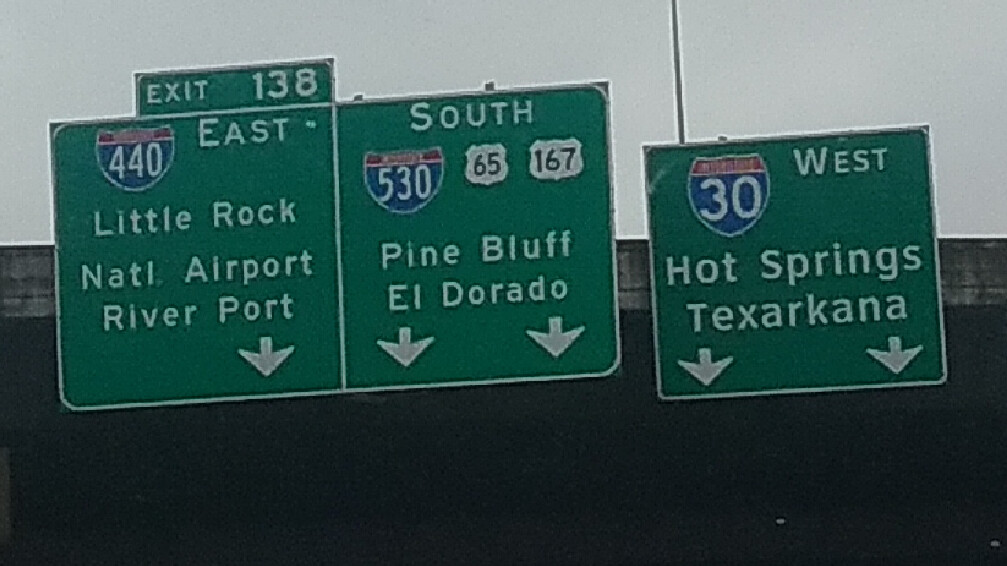In this photograph, an overcast sky looms above, casting a gray hue over the scene. Beneath it, an almost black underside of an overpass extends across the frame as the focal backdrop. Centered prominently are three green highway signs directing traffic flow. The leftmost sign indicates "West Hot Springs Texarkana" with a blue and white Route 30 shield and two white arrows pointing down at separate lanes. The middle sign designates "South Pine Bluff El Dorado" and features Route 530, Route 65, and Route 167 with two white arrows pointing downwards. The rightmost sign reads "Exit 138, Route 440 East, Little Rock National Airport Riverport," accompanied by one white arrow pointing down. Despite the overall low quality of the image, the text on the signs remains clearly visible and legible.